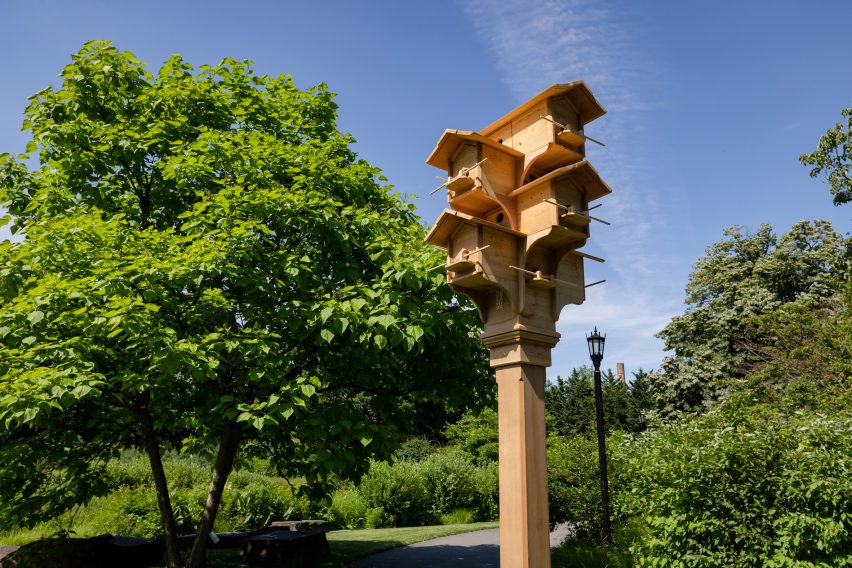In this rectangular photograph taken on a sunny, mostly clear day with a smattering of light clouds in the blue sky, a picturesque outdoor scene unfolds. In the center foreground, slightly to the right, stands an elaborate, beige-colored wooden post adorned with four rows of birdhouses. Each row features two birdhouses, with the total amounting to eight, all stacked in an alternating pattern and pointing in different directions.

The lush background is populated with deciduous trees and bushes, and a few evergreens peek through from the back. Among the greenery, a large tree to the left provides shade for a picnic bench or possible retaining wall, while a concrete path runs through the middle of the scene. To the middle-right background, there is a lamppost, adding to the quaint atmosphere of what appears to be either a park or a spacious yard. The surroundings are rich with green foliage, indicating vibrant summer weather, enhancing the serene, inviting feel of the image.